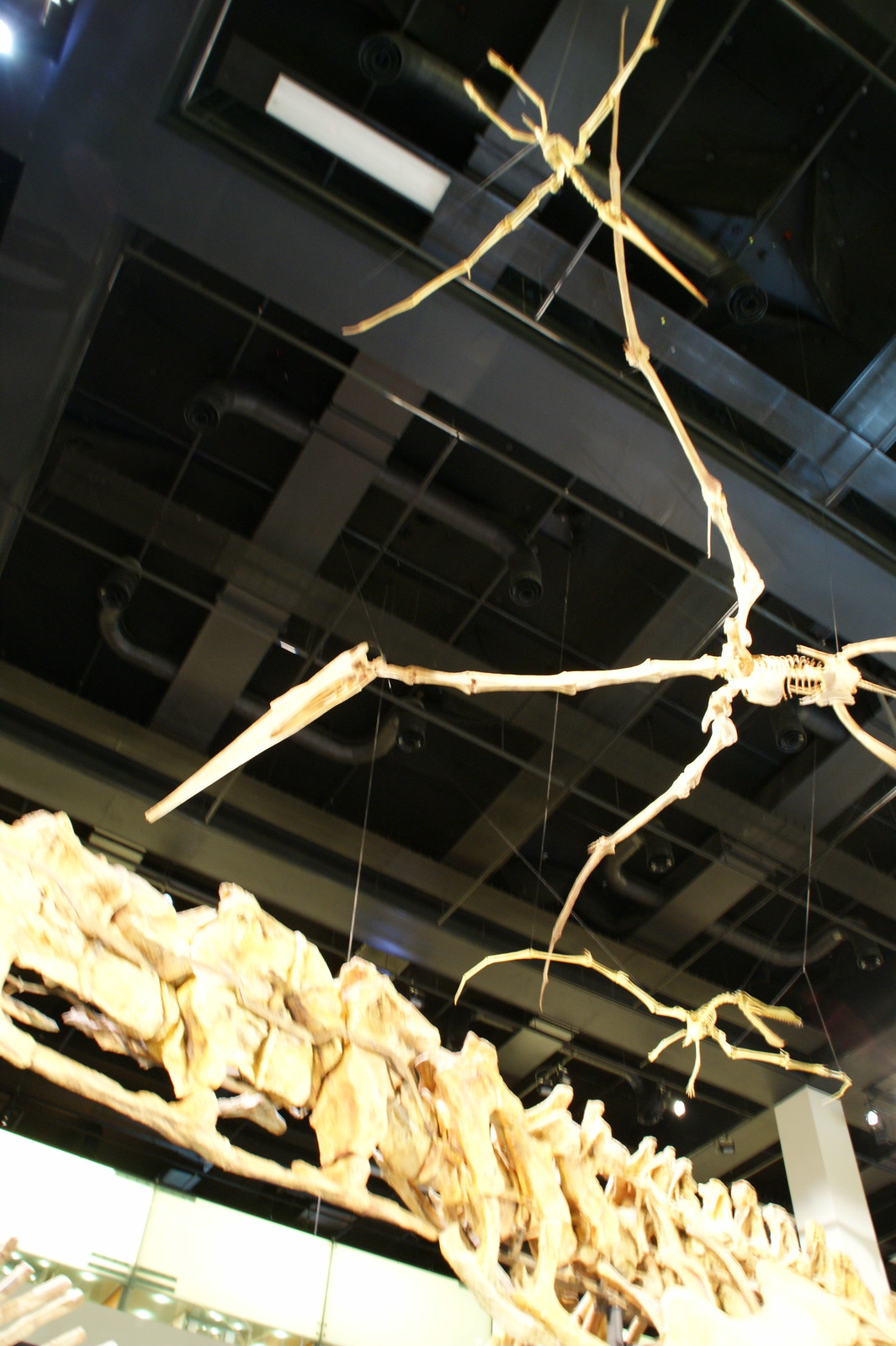The photo captures an upward view in a museum, showcasing an industrial black ceiling structure with numerous bars, girders, and pipes. Suspended from this complex framework are the skeletal remains of three pterodactyls, with their wings spread wide, highlighted by a fluorescent light in the upper left corner. The entire scene is partially covered by glass, accentuating the intricate details of the display. Below the pterodactyl skeletons, a thicker, more robust spine of another prehistoric creature stretches from left to right, though only a portion of this larger dinosaur skeleton is visible. The illuminated glass below this thicker skeleton suggests another exhibit area underneath the current view.